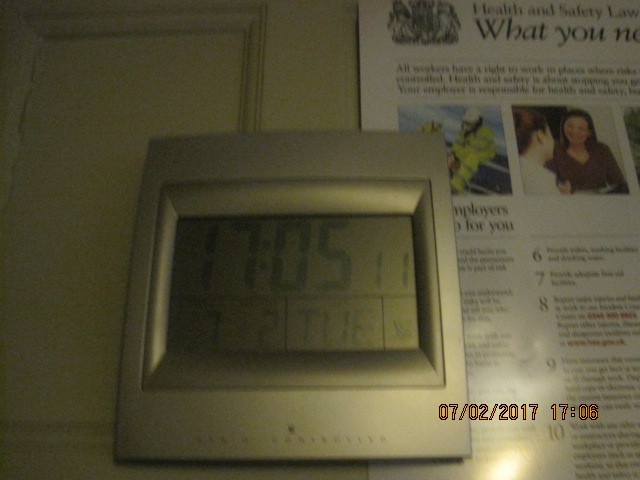This photograph showcases a gray plastic digital clock positioned atop a white, inset-panel cabinet door, accompanied by a partially visible newsletter. The clock, square in overall shape with a rectangular display, prominently shows the time as 17:05. Additional smaller numerals beside the time read "11," followed by "7" and "2" below, and the day "TUE" next to it. The cabinet door, painted white, contrasts subtly with the clock.

The blurred newsletter beneath the clock bears the headline in black text: "Health and Safety Law, What You..." though the rest of the headline is cut off. Despite the unreadable body text, discernible elements include numbered points 6 through 10, along with several images. One photograph depicts firefighters in reflective gear, while another shows two women—one in a white shirt with her hair pulled back, and the other in a dark shirt with shoulder-length hair.

Additionally, the bottom edge of the image is marked with a date and time stamp: "07-02-2017, 17:06."